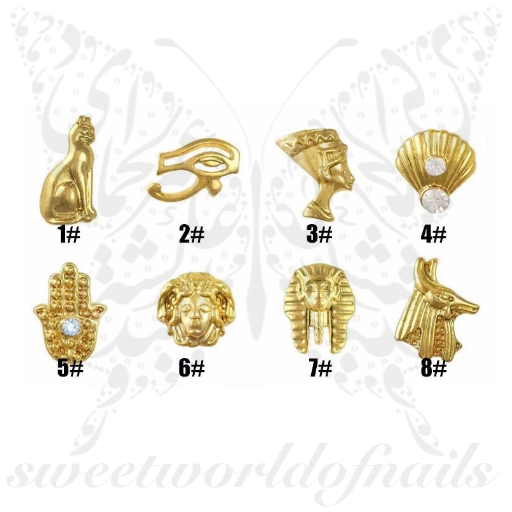This is a horizontal-rectangular image showcasing eight distinct pieces of Egyptian-themed gold jewelry, each labeled with numbers from one to eight. The background features white, textured paper with an indistinguishable, possibly non-English inscription at the bottom. Additionally, a faint gray butterfly and the text "sweet world nails" are subtly visible in the background.

The gold medallions are presented in an orderly fashion:

1. A figure resembling a cat, reminiscent of ancient Egyptian depictions.
2. A hand with a stone embedded in the center, ornate in design.
3. A medallion with an Egyptian symbol or possibly an "evil eye" motif.
4. The depiction of a seashell containing a gemstone.
5. Another hand, this one detailed with intricate gold work and possibly a clock in the middle.
6. An ornate face adorned with flowing golden hair, potentially a deity or figure of significance.
7. The front view of a Pharaoh’s head, complete with traditional headdress.
8. A figure that appears to be a wolf-like creature looking to the right, evoking the image of Anubis in its form.

These detailed, variously shaped amulets exude a rich Egyptian cultural essence, hinting at the available collection that might be ordered.